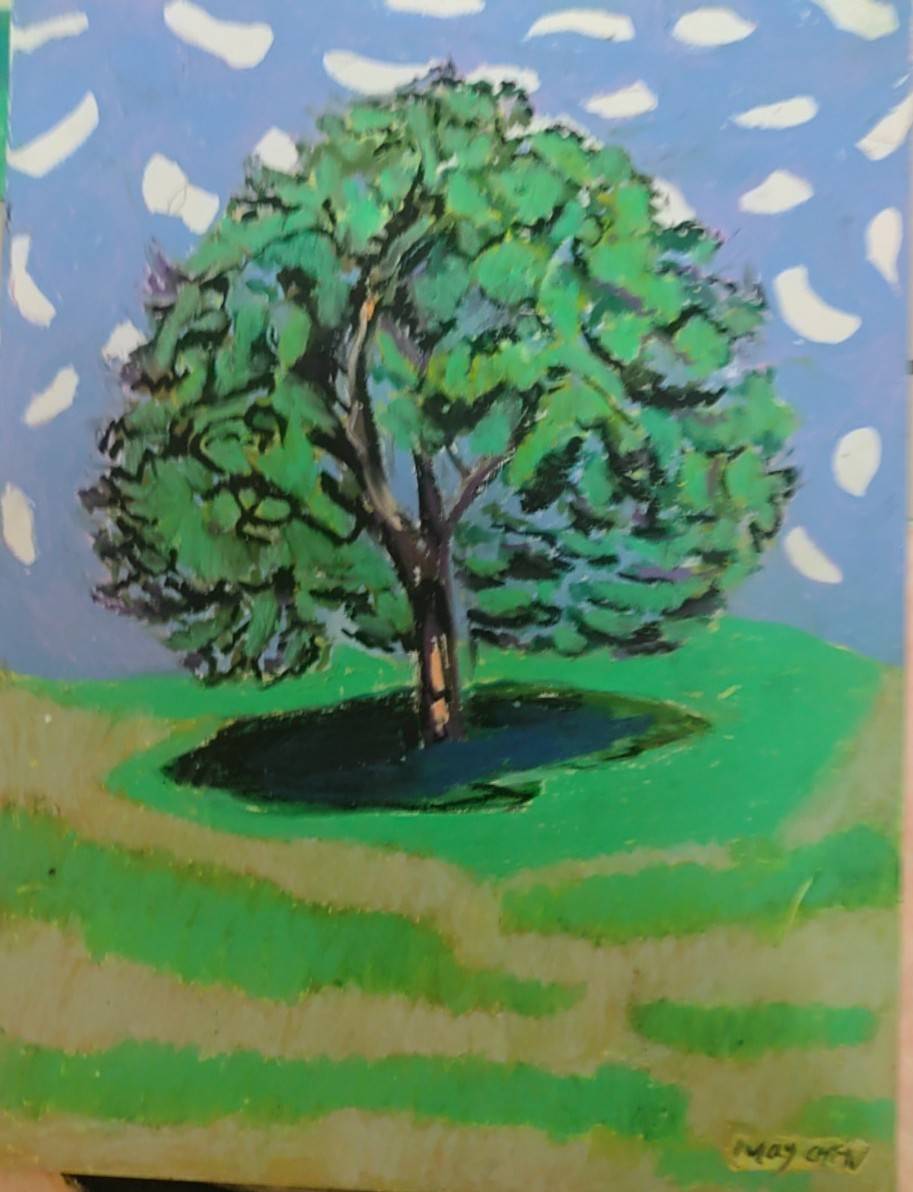This image showcases a slightly blurry artwork, predominantly featuring a large, bushy tree with a slender trunk set against a white background. The background is dotted with small, petal-like shapes intended to represent clouds. The tree casts a substantial shadow beneath its canopy, and scattered green lines vaguely depict patches of grass around the base, with minimal detail. The ground is subtly accented with a lighter brownish hue, suggesting dirt. In the lower right-hand corner, a signature is visible; although the first name is not legible, the last name reads "Chen." This could potentially be a student's mixed-media piece or painting.